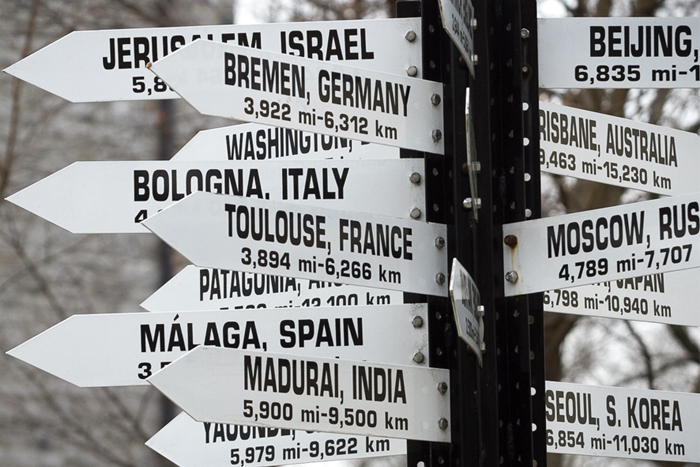The black-and-white photograph captures a tall pole adorned with numerous arrow-shaped signs pointing in various directions, each indicating distances to different countries and cities around the world. At the top, Beijing is prominently displayed, followed by Moscow, South Korea, and further down are signs for Madura in India, Malaga in Spain, Toulouse in France, Bologna in Italy, and a partially obscured sign suggesting Washington. Additional destinations include Bremen in Germany and Jerusalem in Israel. The signs continue with listings for Patagonia, Japan, and Brisbane, Australia. The background features faintly visible trees under a snowy white sky, adding to the stark, monochromatic ambiance of the scene. This signpost, likely located in a central or Middle Eastern region based on the directional indicators, serves as a global mile marker, showcasing how far major cities are, presenting a visually striking and informative landmark.